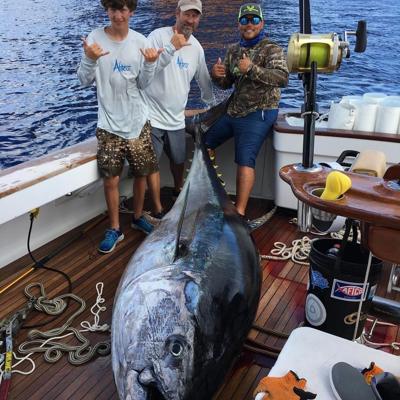This photograph captures a candid moment from a joyful family fishing trip. In the image, three males - two middle-aged men and a teenage boy - stand at the back of a large fishing boat. The serene blue ocean stretches out behind them. The boat features raw stained wooden flooring and painted white sides. The teenage boy, positioned on the left, has curly brown hair and wears a white long-sleeved t-shirt with blue writing and shorts. The two middle-aged men beside him are in white t-shirts with blue lettering and a camouflage-patterned long-sleeved t-shirt, paired with swimming trunks and blue shorts respectively. Two of the men sport ball caps, with one also wearing sunglasses. They are all giving the 'hang ten' hand signal, exuding happiness and pride. At their feet lies an enormous fish, so large it dwarfs the men, leading one to marvel at their remarkable catch or even question the photo’s authenticity. The boat also contains various fishing gear, enhancing the scene's authenticity and charm.